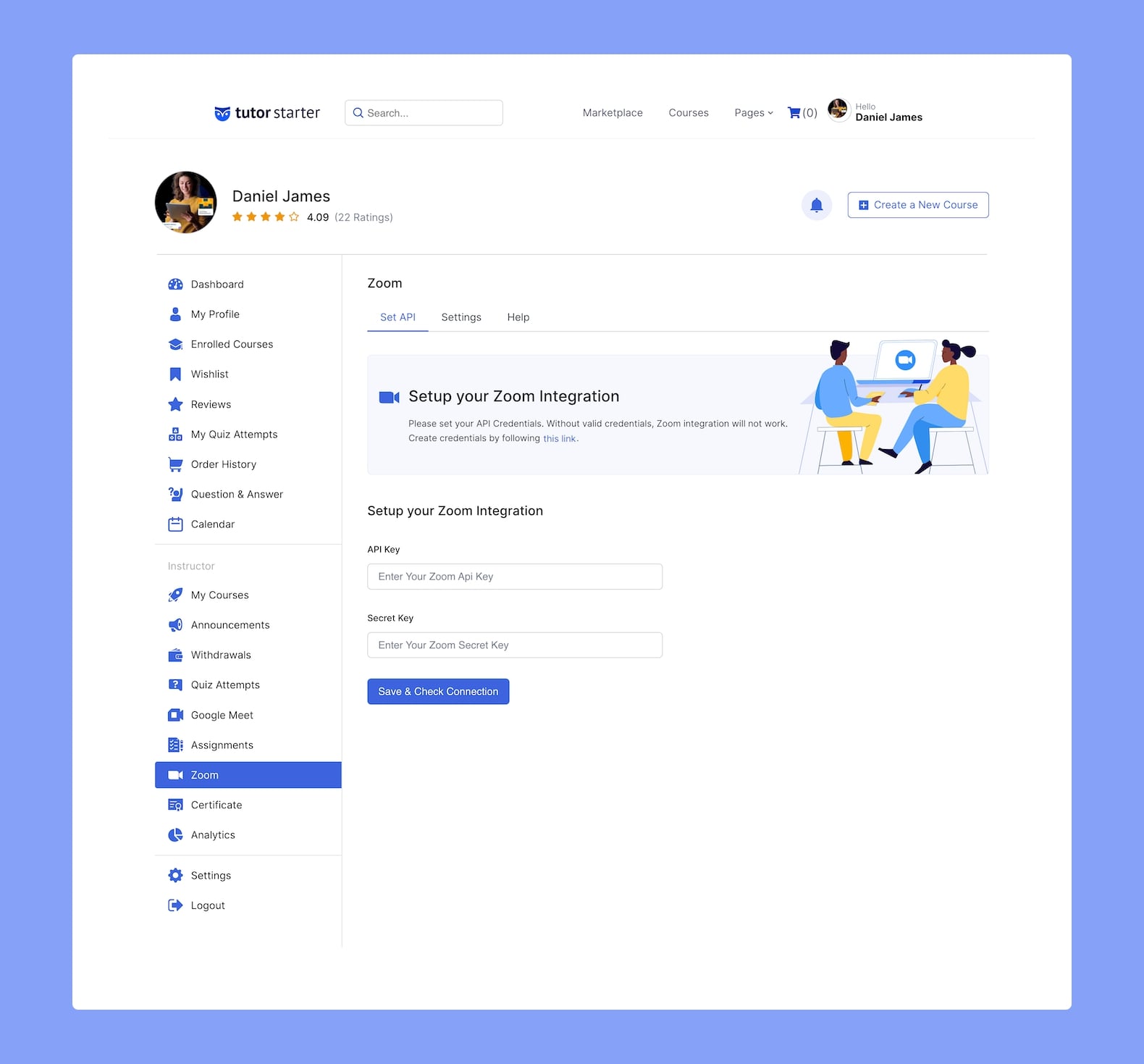Screenshot of an Online Learning Platform Interface

The screenshot appears to be from an online learning platform, displaying a well-organized layout with multiple sections and functionalities. 

At the top of the page, labeled "Tutor Starter," is a navigation bar featuring a search function, links to a marketplace, courses, and pages, as well as a shopping cart icon, which is currently empty. The user profile name displayed is Daniel James, accompanied by a circular avatar of a woman with long hair wearing a yellow top and holding a tablet. The tutor has a rating of 4.09 stars based on 22 ratings.

On the left side, there is a vertical sidebar with a variety of blue icons and categories. The categories listed include:
- Dashboard
- My Profile
- Enrolled Courses
- Wishlist
- Reviews 
- My Quiz Attempts 
- Order History
- Questions and Answers 
- Calendar
- Instructor
- My Courses
- Announcements
- Withdrawals 
- Quiz Attempts 
- Google Meet 
- Assignments 
- Zoom (currently highlighted in blue)
- Certificate 
- Analytics 
- Settings 
- Logout

To the right of the sidebar, detailed information about Zoom settings is displayed. Users are prompted to "Set API credentials" for proper Zoom integration, with detailed instructions and a blue-colored help link. Additional settings and help options are available on the right side. 

A cartoon illustration of a man and a woman sitting in front of a computer displaying the Zoom logo complements the instructions. The man is dressed in a blue top and yellow trousers, while the woman wears a yellow top and blue trousers. Below this illustration are input fields labeled "API Key" and "Secret Key," accompanied by a blue button that says "Save and Check Connection" in white text.